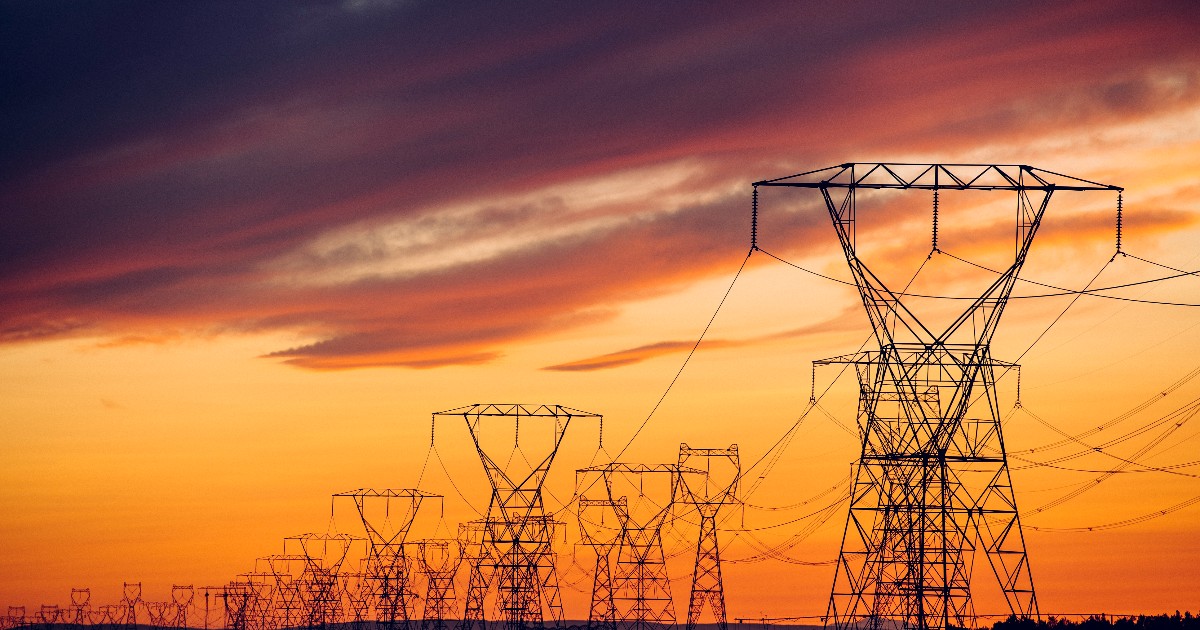This vivid color photograph captures an expansive field of silhouetted metal power line towers stretching horizontally from left to right, with the power lines drooping between them. The scene is set against the dramatic backdrop of a sunset sky that transitions from dark gray and purple-pink at the top, to deep oranges and yellows, and finally to a lighter orange near the horizon. The sky is filled with thick clouds that reflect various hues of gold and gray. Notably, a particularly tall power line tower dominates the right side of the image, while the tops of some trees are visible in the bottom right corner of the photograph. This stunning dusk setting ensures that these structures stand out starkly against the vibrant, multi-colored sky, creating a striking and detailed composition.